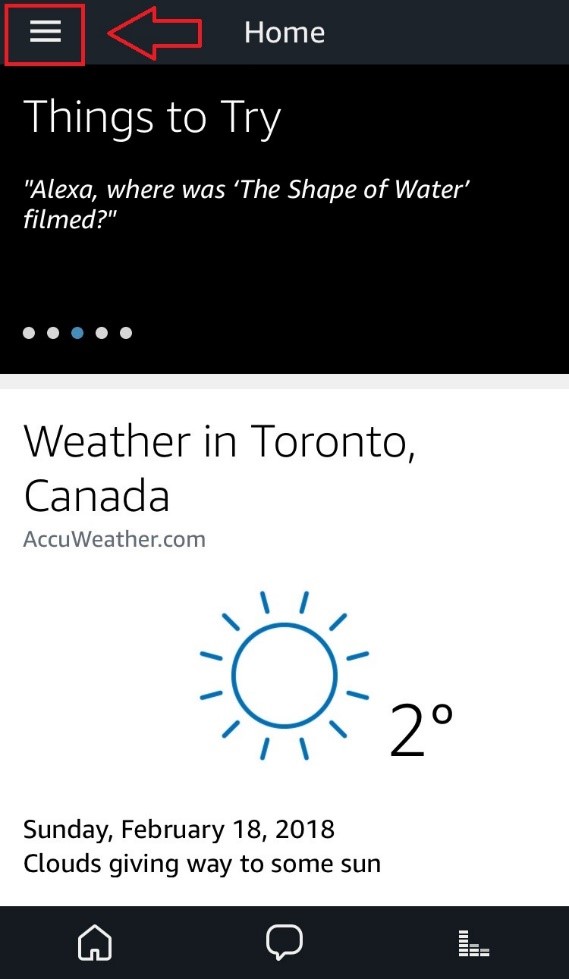The image features a graphical user interface with various sections and elements that cater to user interaction and information display. 

At the top left corner, a white-colored hamburger menu icon is encased in a red square. Adjacent to it, on the right, is a red arrow pointing towards this red square. Continuing to the right is the text "Home" in white, set against a dark gray background.

Directly below is a prompt section that begins with the text "Things to try," followed by a query example, "Alexa, where was The Shape of Water filmed?" Near the bottom left of this area are five small circles. Four circles are white, while the center circle is blue, all set against a black background.

In the middle section of the image, slightly lower, is a weather update for Toronto, Canada, sourced from AccuWeather.com. It includes a blue sun icon, the temperature reading "2°C," and the text "Sunday, February 18th, 2018" with a weather description, "Clouds giving way to some sun," all set on a white background.

Conversely, at the very bottom of the image, three icons are aligned from left to right—a home icon on the far left, a text bubble icon in the middle, and an icon resembling a declining graph on the far right. These icons presumably facilitate navigation and additional functionalities within the interface. 

Overall, the interface uses distinct color coding and clear text labels to enhance usability and visual organization.